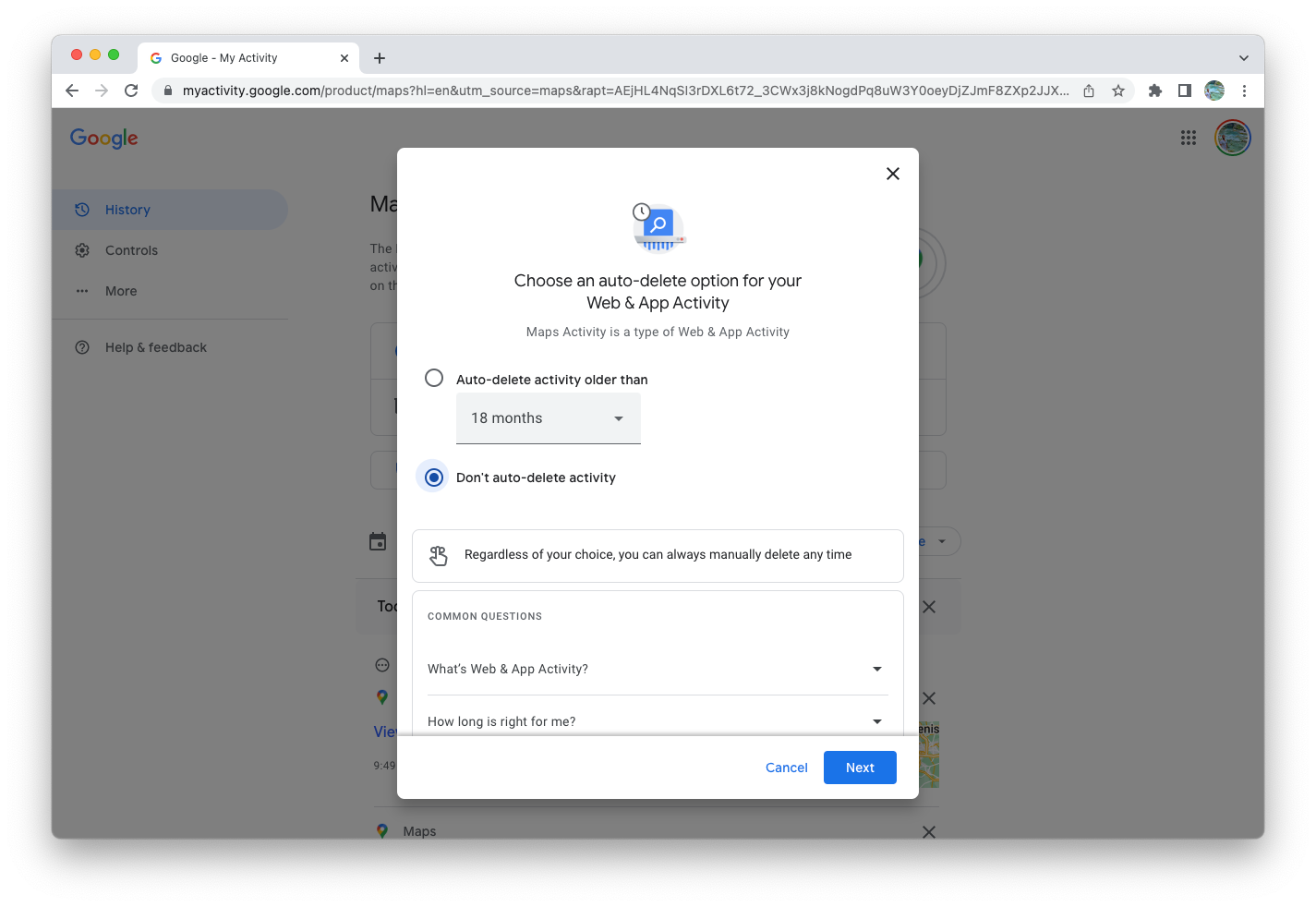The image features a Google "My Activity" page displaying a navigation sidebar on the left with options such as "History," "Control," "More," and "Help and Feedback." Some text in this sidebar is obscured. A prominent white pop-up box is present on the screen, overlaid with an "X" for closing in the upper right corner. At the top center of the pop-up is a blue square icon containing a magnifying glass and a clock in the upper left corner. The header under the icon reads, "Choose an auto-delete option for your web and app activity."

The main content of the pop-up explains that "Maps activity is a type of web and app activity," followed by two selectable circles. The first option, labeled "Auto-delete activity older than 18 months," is not selected. The second option, already selected and highlighted in blue, reads "Don't auto-delete activity." Below this, there's a note stating, "Regardless of your choice, you can always manually delete any time." Further down, frequently asked questions are listed, including "What is web and app activity?" and "How long is right for me?" At the bottom of the pop-up, there are two buttons: a grey "Cancel" button and a blue "Next" button.